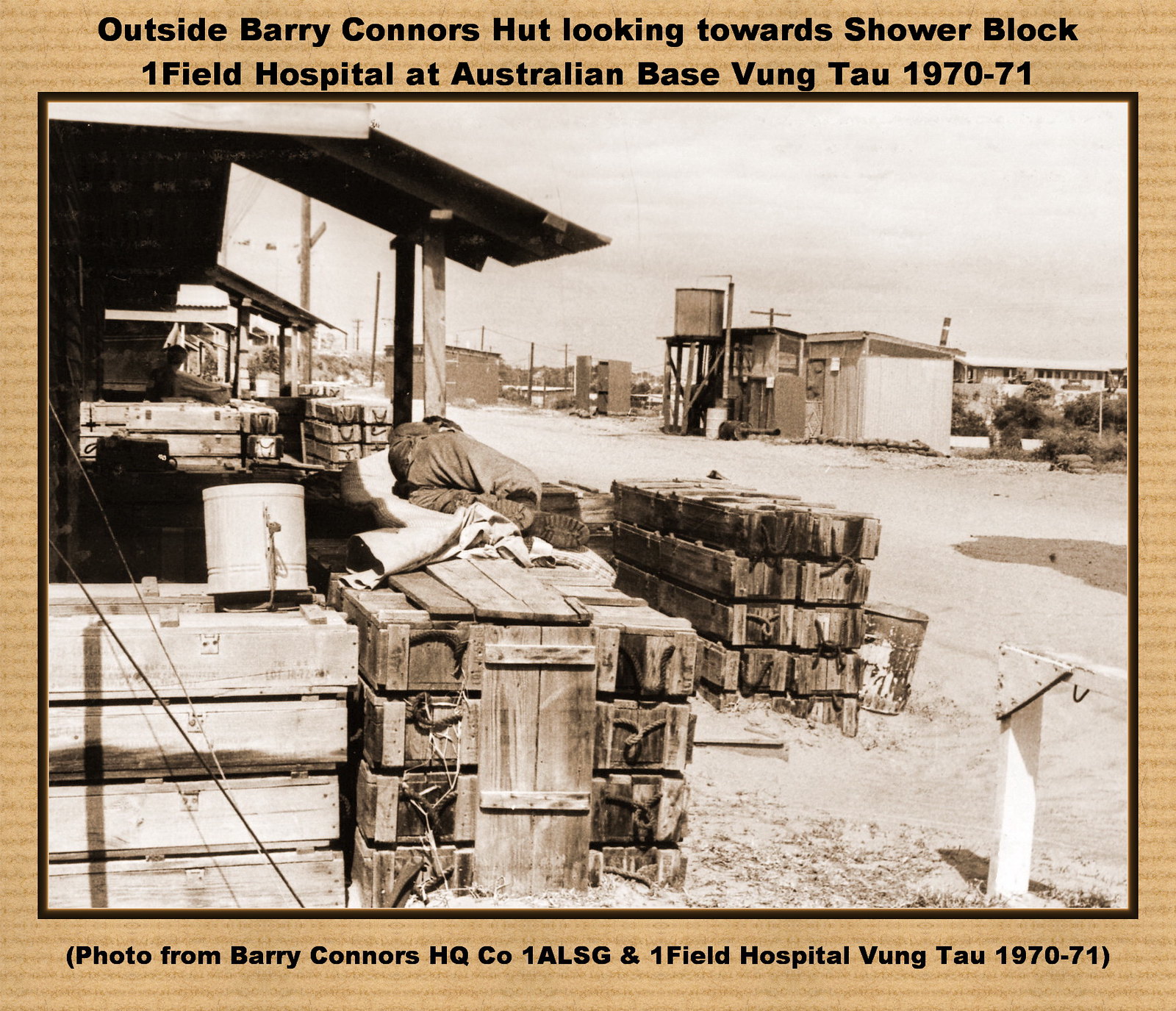This sepia-toned, black-and-white photograph, framed with a tan border, captures a segment of a military base, likely from the 1970-71 period, at the Australian Base in Vung Tau. The image foregrounds numerous wooden crates and barrels, some stacked against a fence, with a bucket perched on one of the crates. The scene includes an array of outbuildings and shacks, evoking the appearance of a small, perhaps deserted, village. To the right, a white building and a water tower with a container at the top are visible, with shrubbery encroaching from the background. The left side features more overhanging structures sheltering additional supplies. The sky is an empty expanse of white. At the top of the photo, text reads, "Outside Barry Connors Hut, looking towards Shower Block, Onefield Hospital at Australian Base, Vung Tau, 1970-71," and at the bottom, "Photo from Barry Connors Headquarters Company, 1ALSG, Onefield Hospital, Vung Tau, 1970-71."